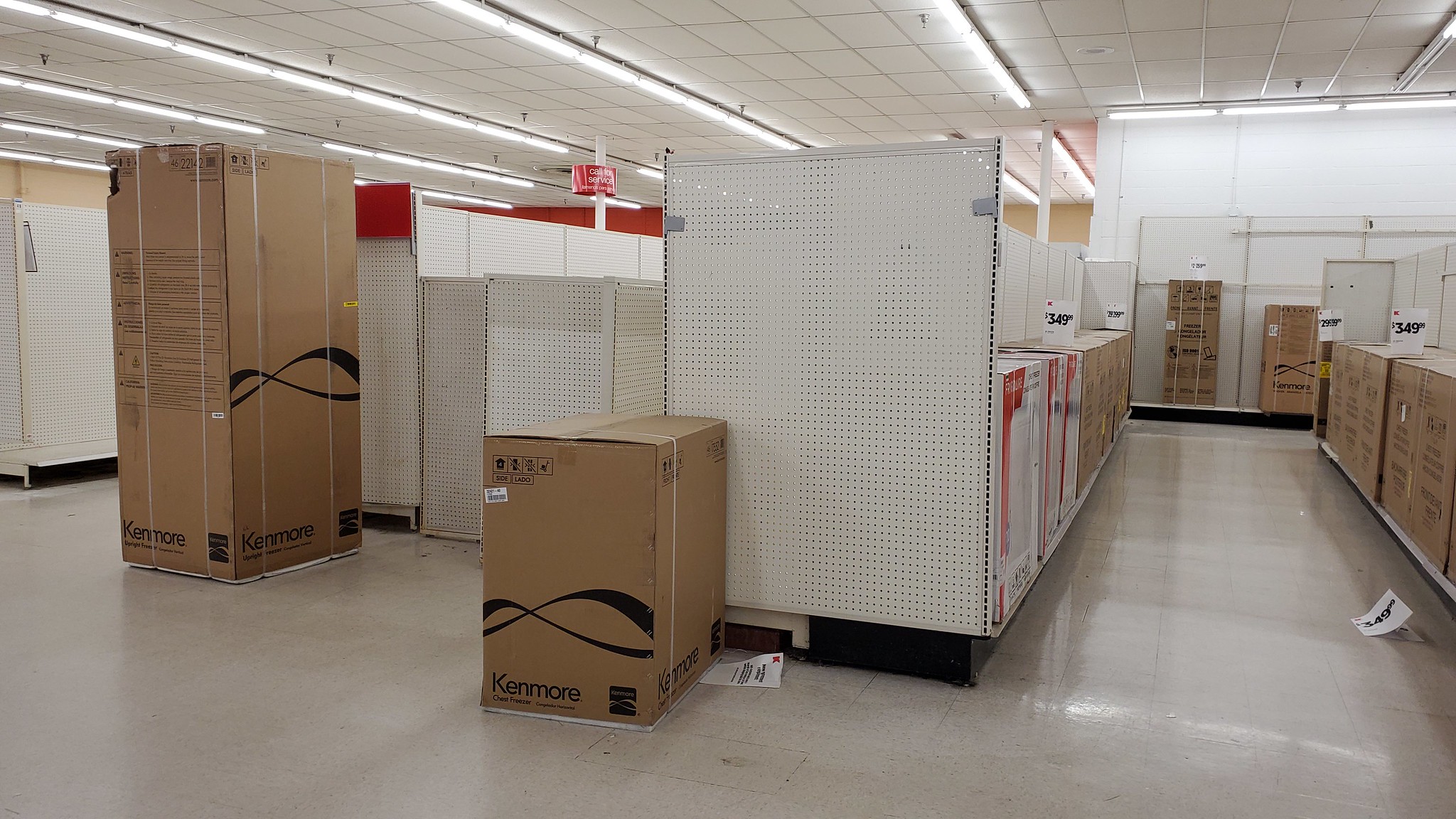This detailed photograph depicts the interior of what appears to be a Kmart store in a state of clearance or closure. The floor is tiled in light beige, extending uniformly throughout the scene, and the ceiling consists of a grid of white tiles embedded with fluorescent lights mounted on gray tracks. These lights are vividly bright and run horizontally across the ceiling in rows.

Dominating the center of the image are white shelves, most of which are largely empty or host a few brown cardboard boxes. In particular, on the left side, there are two prominent brown boxes. The first box, positioned on the lower left side, displays the word "Kenmore" in black writing at the bottom left corner. To the left of this, closer to the edge, stands a taller brown box with vertical strapping and "Kenmore" also marked in black text.

Further into the background, more cardboard boxes with a similar appearance, some featuring a hard-to-see white and red design, are scattered on the shelves. Several white signs with black text, displaying prices like $349.99 and featuring a red "K", can be seen attached to the shelves, reinforcing the possible Kmart connection. The sparse stocking and evident labeling suggest that the store is in the process of clearing out its remaining inventory.